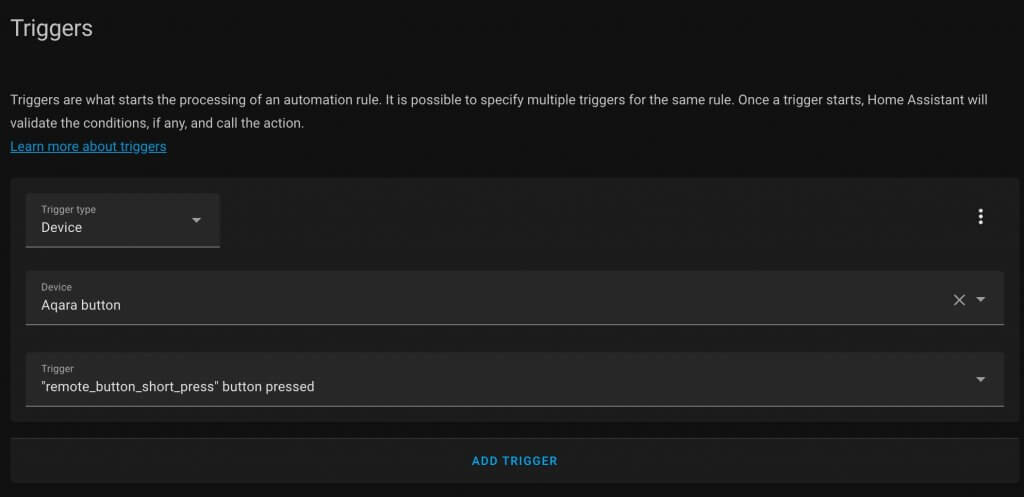**Detailed Caption:**

The image displays a screenshot of a Home Assistant interface on a device with a black background, showcasing a page dedicated to setting automation triggers. The title "Triggers" is prominently displayed at the top, followed by an informational section explaining that triggers initiate the processing of an automation rule. Users can specify multiple triggers for the same rule. When a trigger activates, Home Assistant will check the conditions, if any, and execute the specified actions. Below this explanation, there's a blue hyperlink titled "Learn more about triggers."

The main content of the page features three primary clickable fields:
1. **Trigger Type**: Currently set to "Device," with a drop-down arrow indicating it can be changed.
2. **Device**: Indicated as "Aqara button."
3. **Trigger**: Described as "Remote button short press, button pressed."

At the bottom of the interface, there is a prominent blue button labeled "Add Trigger," which suggests that users can add more triggers to their setup. The overall layout indicates a sophisticated and detailed system that likely requires a good understanding of Home Assistant terminology to utilize effectively.